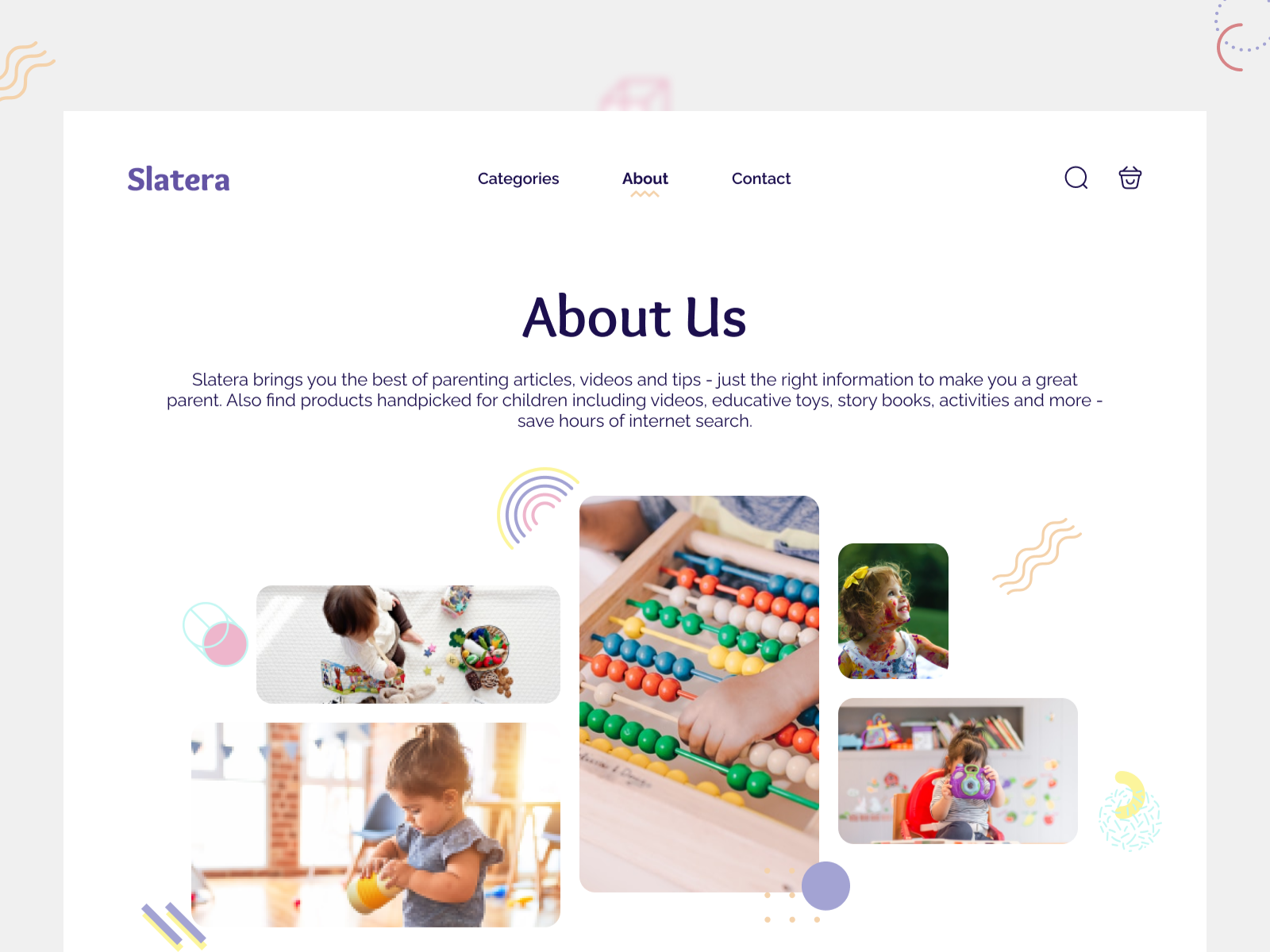The image portrays the homepage of a website called Slatera, emphasizing parenting resources. The top navigation bar includes options like "About" and "Contact," accompanied by a search bar and a cart icon. The About page prominently displays the message: "Slatera brings you the best of parenting articles, videos, and tips, providing just the right information to help you become a great parent. Also, explore handpicked products for children, including educational videos, toys, stories, activities, and more. Save hours of internet search with Slatera."

The website features a clean design with a white background and dark blue or black text. The page is visually enriched with photos of children engaged in various activities. There are five distinct images: one of a child holding a toy camera, another of a child covered in paint, a third showcasing beads on a counting toy, and a girl holding a plastic object. The vibrant colors in the photos include red, blue, yellow, green, pink, brown, and purple, adding a lively and engaging touch to the site.